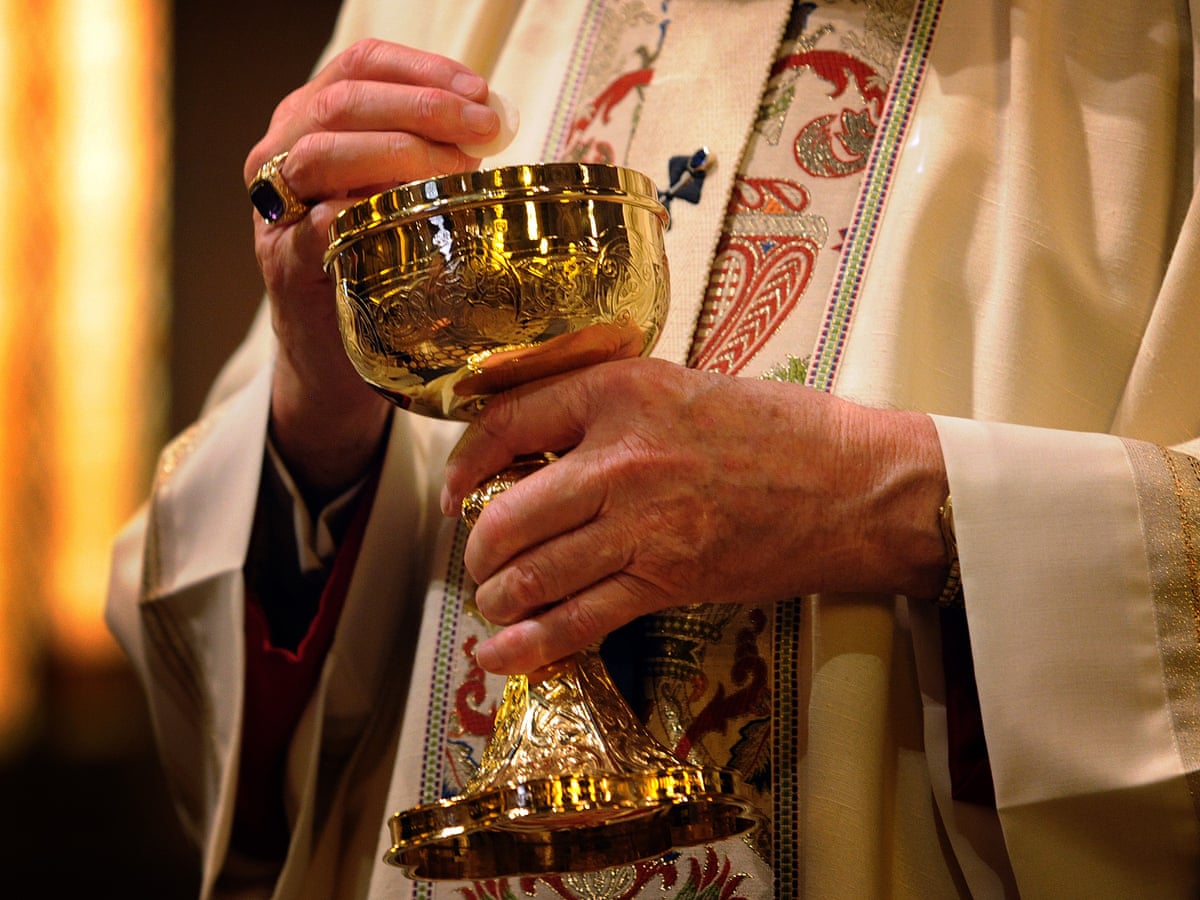This detailed image depicts a priest during a religious ceremony, specifically communion. The priest is holding an ornate gold chalice with a flat, intricately designed base in his left hand, and a communion host in his right hand. He is wearing traditional mass vestments, which include an off-white robe and an elaborately embroidered stole with vivid red, green, and some purple patterns reminiscent of Slavic or Eastern European designs. His right ring finger is adorned with a gold ring set with a large purple jewel. The priest's robe reveals a red-sleeved jacket, suggesting additional layers of religious garments underneath. In the background, a blurry stream of light filters through a window, and a yellow curtain is visible on the left side of the frame. The priest’s hands show signs of aging, with visible veins and wrinkles, adding to the solemnity of the scene.